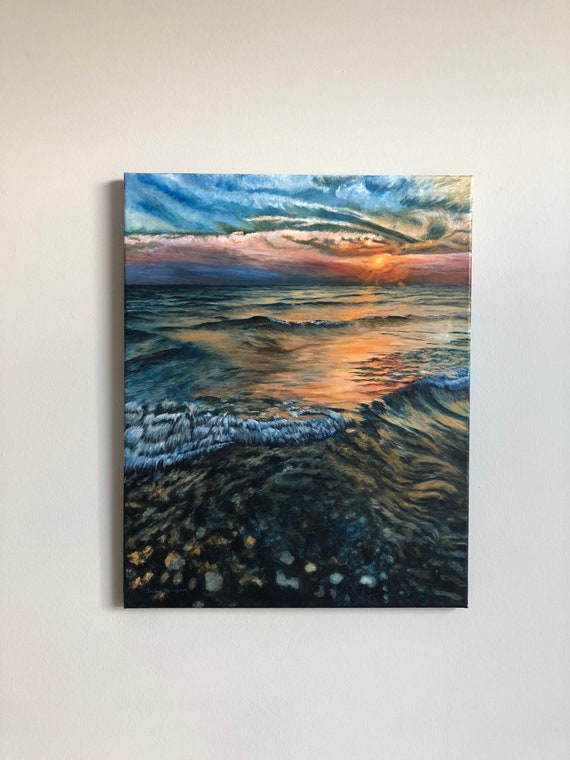This photograph captures a striking painting of a vivid seacoast at sunset. The artist's stylized brush strokes are prominent, lending a textured and dynamic feel to the scene. The composition features a rugged rocky coast protected by a meticulously detailed gray stone retaining wall. Beyond the wall, the vibrant turquoise sea exhibits rolling and rippling waves, which catch the warm orange reflectance of the setting sun. The sky, an unusual yet captivating blend of pink hues with blue and gray clouds, adds to the overall drama of the scene. The clouds themselves are artistically rolled and riffled, enhancing the stylized aesthetic of this captivating seascape.